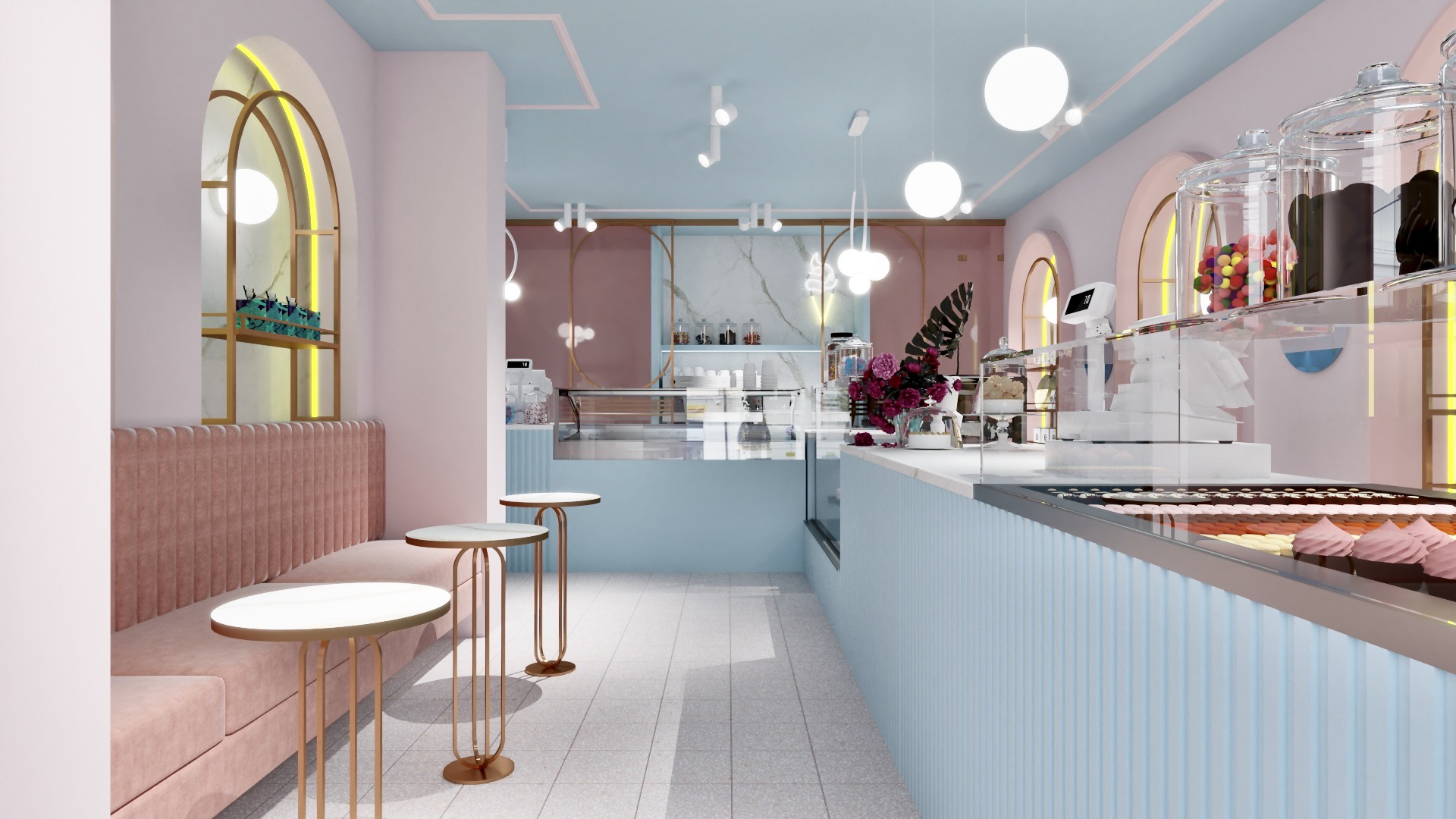The image depicts a brightly lit, 3D-rendered pastry shop or ice cream parlor adorned in light pastel colors. To the left, a section of the shop features a pink couch set against a pink wall, accompanied by small white tables for customers to enjoy their treats. Above the couch, shelves hold various items, adding to the room's cozy atmosphere. On the right, the main counter area houses jars filled with candy, gumballs, and cookies, with a lower section showcasing a glass case for displaying ice cream and cupcakes topped with pink icing. The counter itself is light blue with a white countertop, and the cash register is located at the far left corner. The walls are painted in shades of peach, mauve, and a bright off-white pinkish hue, while the ceiling is light blue with integrated lighting. Completing the scene, a neon sign shaped like an ice cream cone hints at the shop's offerings, emphasizing its dual role as an ice cream and pastry shop. Additionally, flowers decorate the counter, enhancing the overall charming and inviting ambiance.